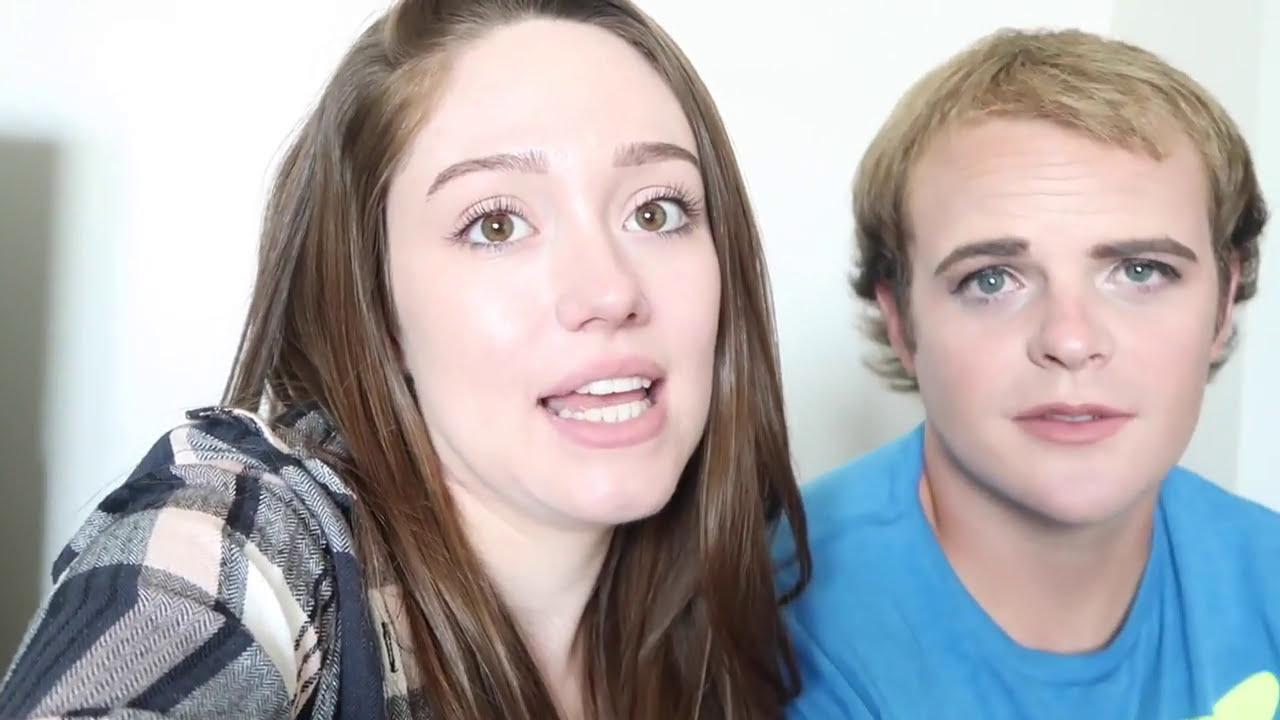This horizontal rectangular photograph features a close-up shot of two Caucasian individuals, a woman on the left and a man on the right, set against a blurry, predominantly white indoor background with the edge of a doorway visible on the far left. The image appears to be a selfie, capturing them from just below the shoulders up. 

The woman, who is situated on the left, has long, straight brown hair parted at the side. She is wearing a black and white, or potentially blue and gray, plaid shirt, which is only visible from her right shoulder up to just under her neck. She has wide brown eyes, long eyelashes, and brown eyebrows. Her mouth is open, revealing her white teeth and a hint of her tongue, as though she is speaking. She is wearing light pink lipstick and has a clear complexion.

Next to her, on the right, is a man with short, blondish-brown hair that darkens near his ears. He has brown eyebrows and striking blue eyes. He is dressed in a white crew-neck T-shirt, although earlier descriptions mentioned a blue shirt, suggesting there may be some discrepancy in color perception. His mouth is slightly open, showing a bit of his teeth, as if he is about to speak or has just finished speaking. Both individuals appear relaxed, engaging directly with the camera.